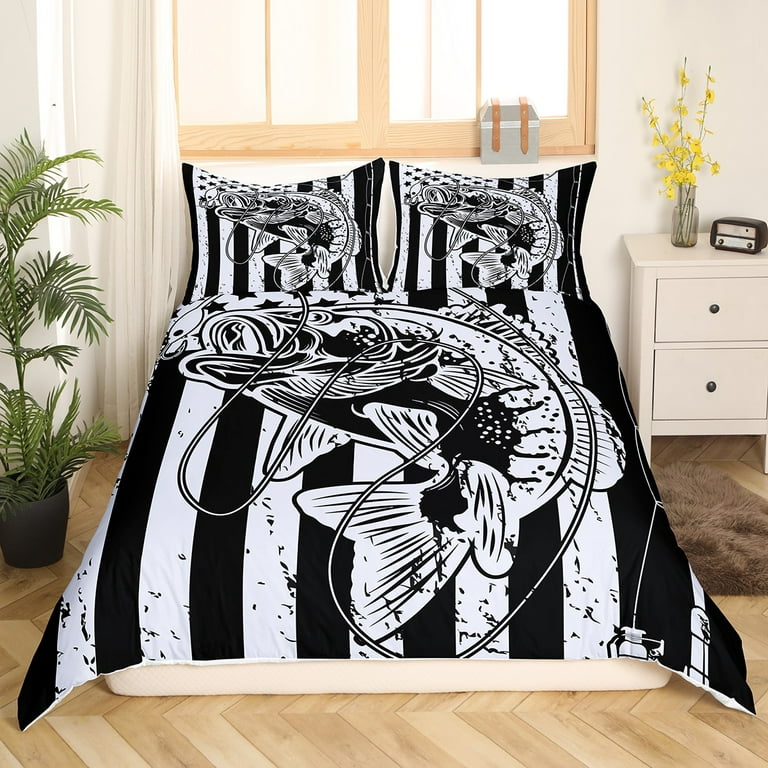The image depicts a spacious, crisply clean bedroom centered around a double bed adorned with a striking black and white comforter and matching pillowcases. The bedding features a bold design of a bass fish with a fishing lure, spanning almost the entire coverlet and replicated on the pillows. The room's floor boasts a distinctive V-pattern wood grain, accentuating the natural aesthetics. To the right of the bed, a white-topped nightstand hosts an alarm clock and a vase with delicate yellow flowers, resting on a small rug. On the left, a four-foot tall fern tree stands in a black pot, adding a touch of greenery. Behind the bed, a wood grain trim window allows natural light to enhance the calming, minimalist ambiance.